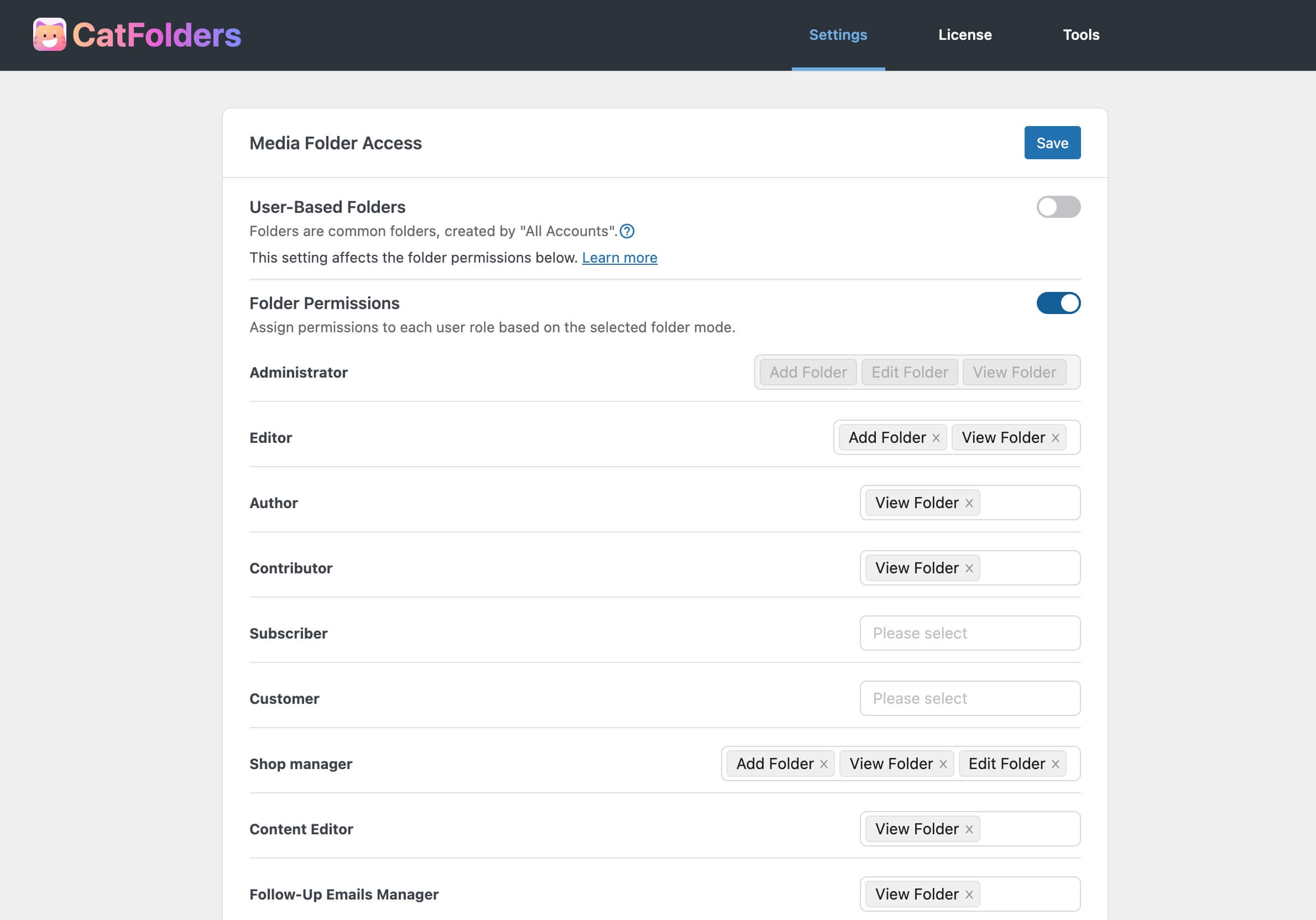In the presented image, a stylized rectangular interface is prominently featured, with a sleek black border on the top portion. Within this black border, a vibrant and colorful icon, which transitions from orange to blue, is displayed. Adjacent to this icon, in similarly colored text, it reads "Cat Folders." Below this section, against a gray background, lies a centrally-positioned white rectangle that contains structured information.

The interface is divided into several organized sections. Below the initial colorful title, "Cat Folders," there is a spaced-out list including "Settings," "License," "Tools," and other elements. The text "Media Folder Access" is prominently mentioned, followed by some spacing and a blue button labeled "Save and Write."

A detailed paragraph explains "User-Based Folders" as folders commonly created by all user accounts. It notes that this setting affects the folder permissions listed below. Associated with this section is a "Learn more" link, alongside a question mark icon within a circle; however, this feature appears to be turned off.

The subsequent section, labeled "Folder Permissions," offers options to assign specific permissions. This is intended to be based on user roles or the selected folder mode, which in this instance is turned on.

The image then elaborates on different user roles, starting with "Administrator," which shows three shaded-out bars indicating its settings. Following this, roles such as "Editor," "Author," "Contributor," "Subscriber," "Customer," "Shop Manager," "Consent Editor," and "Follow-Up Emails Manager" are also listed, providing a comprehensive look at the hierarchical permissions model within this interface.